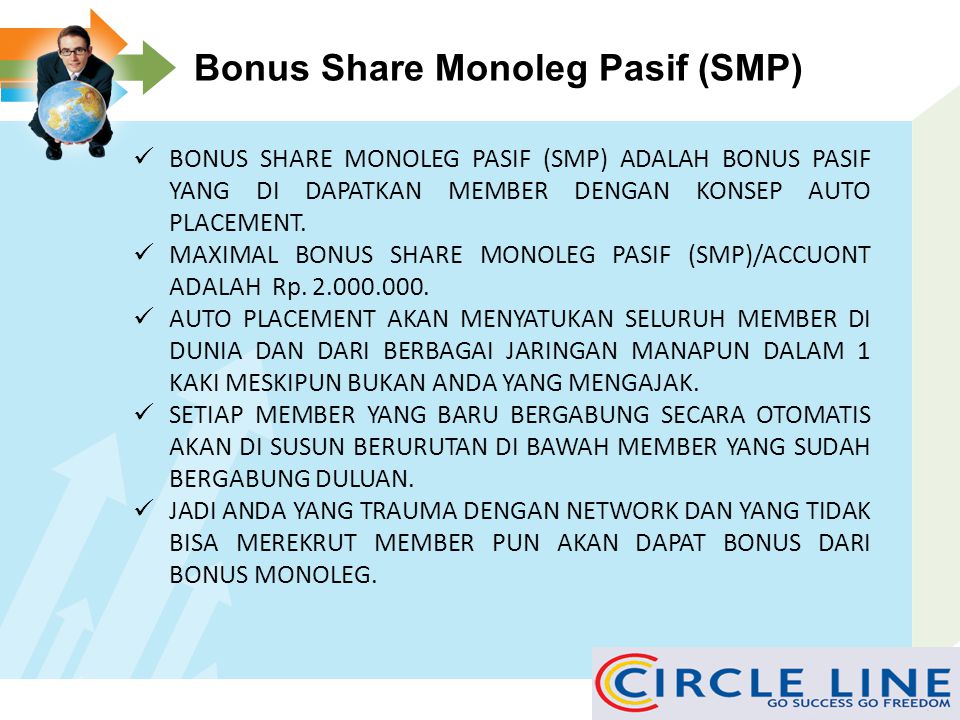The rectangular advertisement features a white header with three right-pointing arrows in the top-left corner—orange on top, green in the middle, and blue at the bottom. Positioned in front of these arrows is a Caucasian man kneeling, dressed in a black suit and jacket, and holding a globe. To his right, bold black text on the white background reads, "Bonus Share Monoleg PASIF (SMP)." Below this, a white beveled border encloses text on a light blue background, with five check marks aligned vertically on the left side. The text, a mixture of languages, includes phrases like "Bonus Share Monoleg PASIF" and "Adala Bono PASIF, Yang Di Dapatkan Member Dangan Concept Auto Placement." In the bottom right corner of the image, a gray rectangle with blue text proclaims, "Circle Line, Go Success, Go Freedom." Adjacent to the word "Circle," a larger gold 'C' is overlaid with a red 'C'.